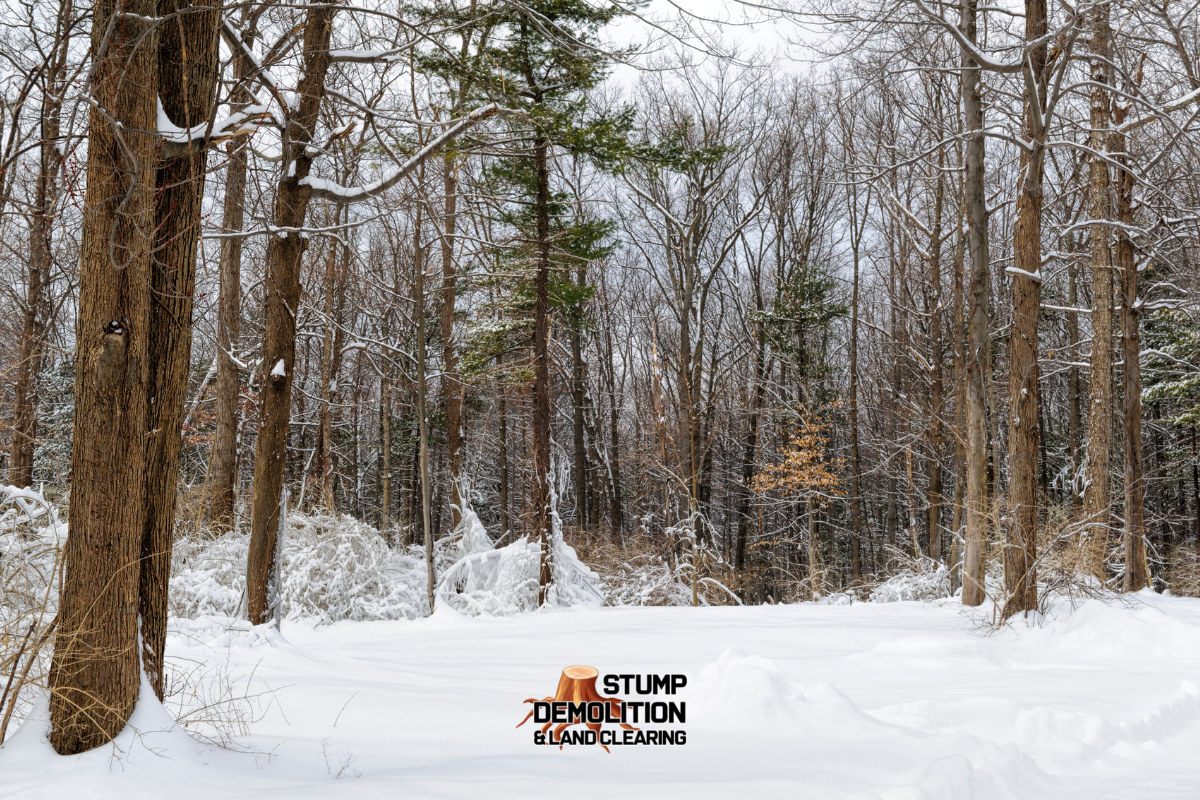This is a color, landscape-oriented photograph of a serene winter scene featuring a snow-covered field and a dense, barren forest in the background. A blanket of white snow, approximately five to eight inches deep, stretches across the entire foreground from left to right. On the left side, a few brown tree trunks emerge from the snow, while on the right, the expanse remains undisturbed and creates a sense of open space. The background is dominated by a densely packed thicket of tall, deciduous trees, devoid of leaves, with a few green pine trees interspersed among them. A light blue sky peeks through the upper parts of the trees, adding a touch of color to the otherwise monochromatic setting. Near the bottom center of the photograph, there is a logo featuring a cut-down tree trunk with exposed roots, alongside the black text "Stump Demolition and Land Clearing" arranged in two lines, suggesting that the visible clearing in the snow is the result of the company's work.